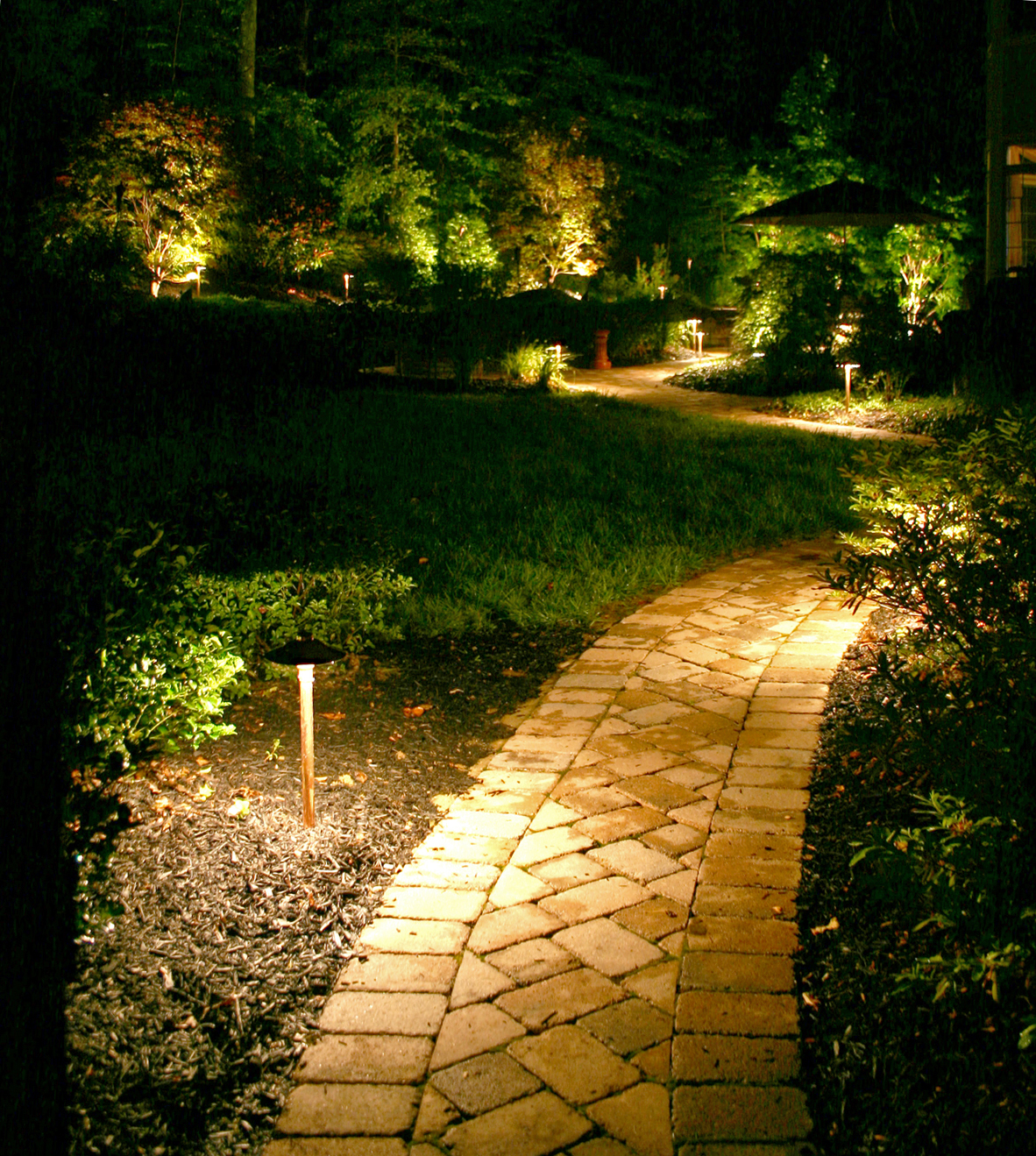The image captures a serene nighttime scene of a curving brick pathway winding through a garden. Starting from the bottom center of the photo, the path arcs to the right, bordered by lush bushes and patches of soil. Small LED garden lamps on tiny poles, emitting a warm yellow glow, line both sides of the walkway, illuminating the path and casting light onto the surrounding greenery. To the left of the path lies a grass field intermittently dotted with bushes, and in the background, the path disappears behind a patio adorned with an umbrella. Tall green trees, including some firs and others with red flowers, form a picturesque backdrop under the dark night sky.